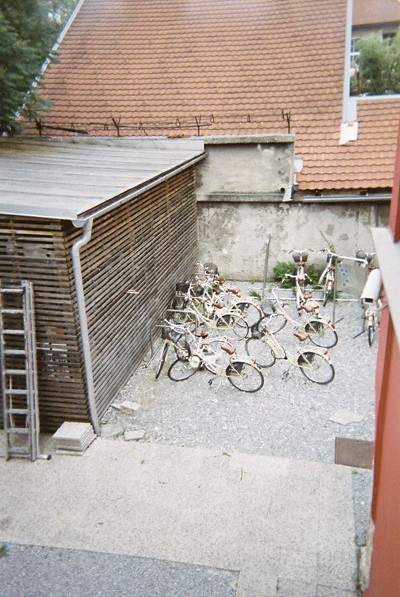The image captures an outdoor scene, seemingly on the roof of a building or an enclosed yard. Dominating the foreground is a smaller, rectangular wooden structure with a tin roof, adorned with lines across its surface and featuring a storm drainage pipe. A silver ladder leans against this building on its right side. On the ground, which consists of a mix of concrete and gravel, rests a dozen white bicycles scattered in various positions. Some bicycles with white seats and red trim are propped against the concrete back wall, others align towards the wooden building, with one notably resting against the structure's right side. Adjacent to the wooden building, there is an imposing reddish-orange slope-roofed structure, adding to the layered architectural elements of the scene. The background reveals shingles from the overarching roof, while trees frame the sides, providing a natural contrast to the man-made elements. Additionally, patio stones appear stacked near the ladder, hinting at ongoing or unfinished work.